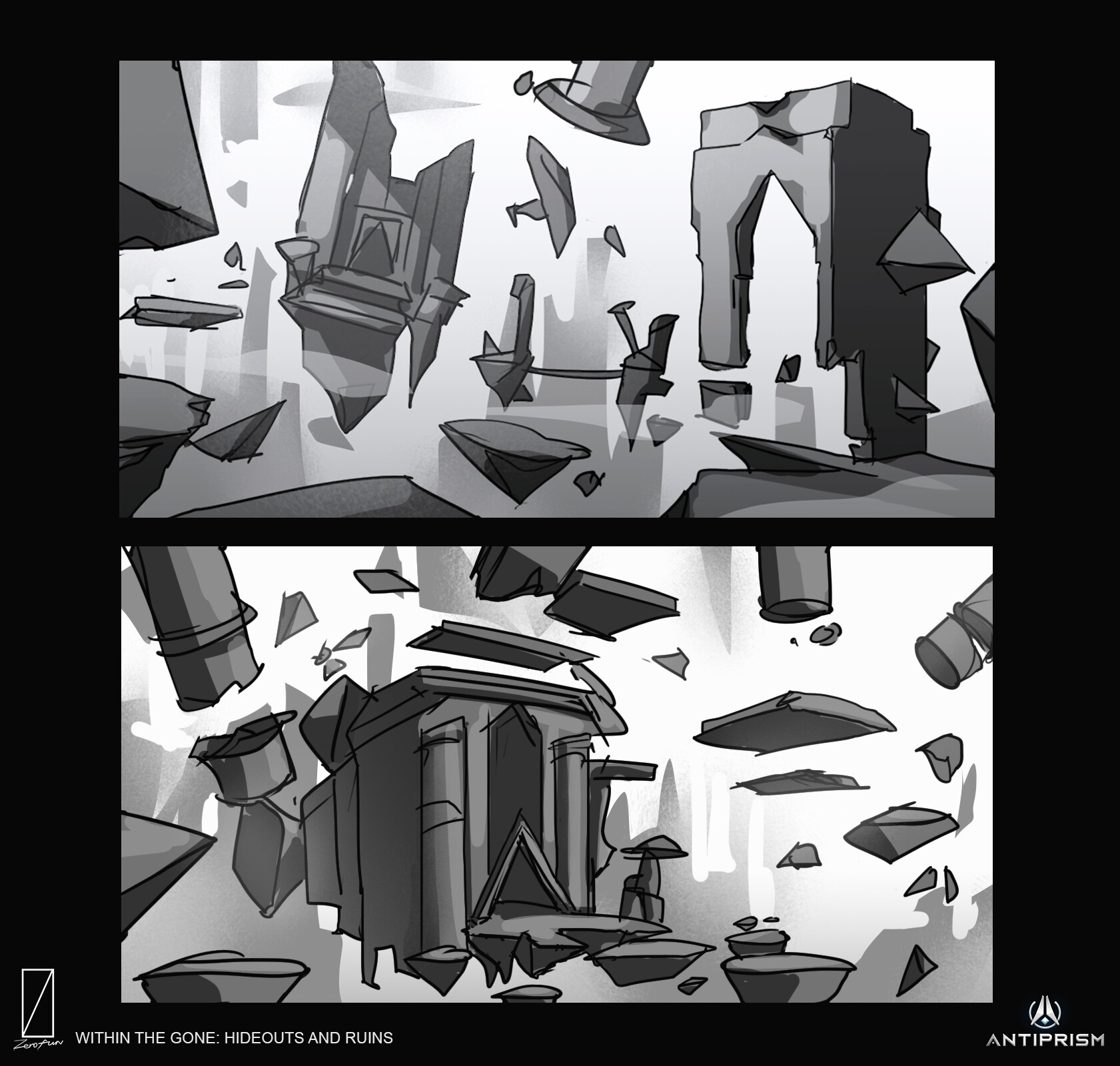The image consists of two computer-generated panels on a black background, arranged with one rectangular panel at the top and another at the bottom. Both panels feature detailed, black and white sketches of a fragmented building, with various pieces floating in midair. The debris includes broken pillars, detached platforms, and an arched doorway, among other architectural elements, all rendered in shades of gray. The columns appear to be the only parts somewhat intact, while the rest of the structure appears shattered and dispersed. The top-left corner of the image contains the text "within the gone, hideouts and ruins," and the bottom-right corner reads "antiprism." The stark, monotone aesthetic and the depiction of floating ruins evokes a sense of desolation and surreal disintegration.